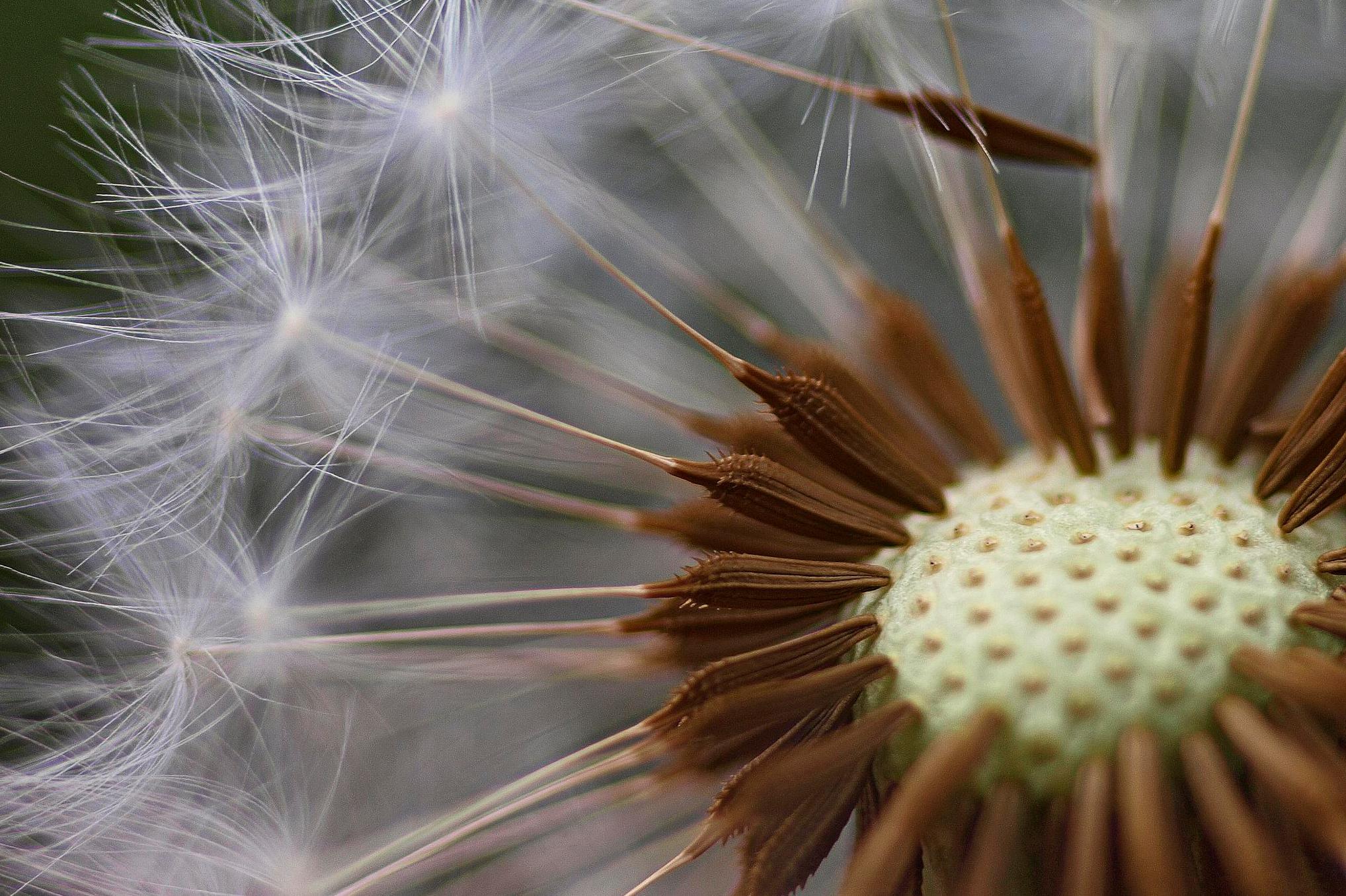This is an incredibly detailed close-up photograph of a dandelion. The central part of the flower is a pale cream or light yellow hue, adorned with numerous dispersed cream-colored dots, resembling tiny beads. Approximately 20 slender, light brown cylindrical stems, resembling reeds, extend from this central orb. These stems culminate in delicate white, feathery structures—those iconic wispy florets that detach easily when blown upon. The intricate composition highlights the seemingly precarious attachment of each fluffy seed to its stem, epitomizing the dandelion's ephemeral nature. The image's tight framing excludes any background details, focusing entirely on the intricate details of the dandelion's structure.